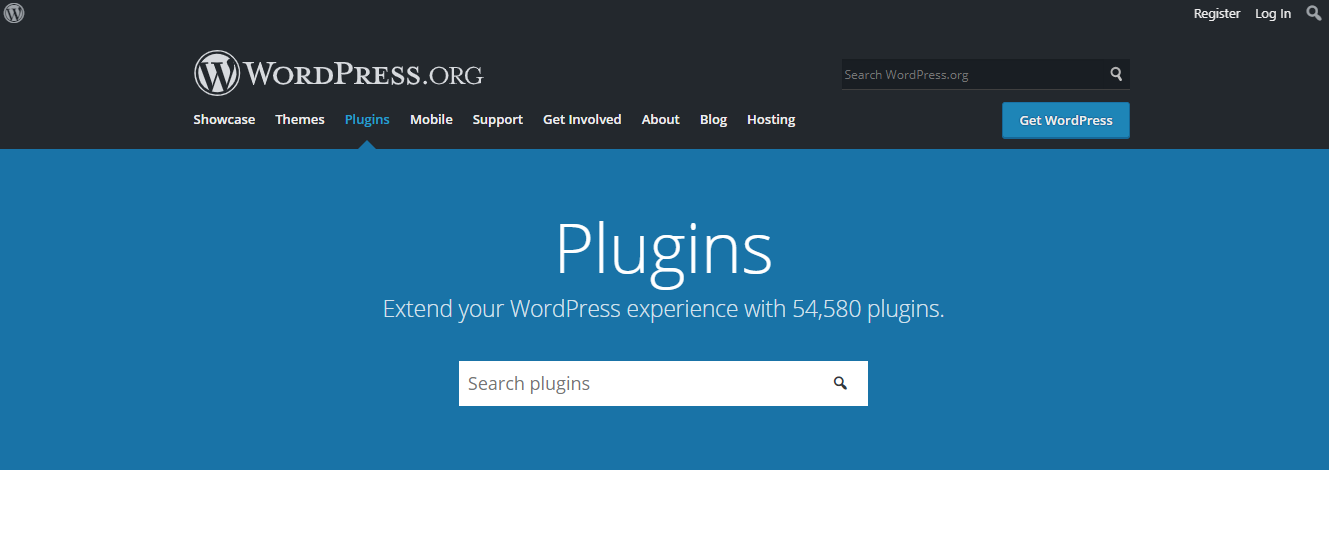The top section of the image features a black banner with "wordpress.org" prominently written in white, positioned towards the middle-left. Directly beneath this banner is a horizontal navigation menu containing links to sections such as Showcase, Themes, Plugins, Mobile, Support, Get Involved, About, Blog, and Hosting. 

On the upper right corner of this navigation bar, there are additional links for Register, Login, and a Search function. Next to these links is a search bar labeled "Search wordpress.org."

Below this navigational area, a prominent blue section spans the page, highlighting the "Plugins" section. The word "Plugins" is displayed in the largest font on the page. Underneath this heading, there is a line of text stating, "Extend your WordPress experience with 54,580 plugins." 

Another white search bar is located below this statement, labeled "Search plugins." The page predominantly features teal blue, black, and white colors. A noticeable blue button labeled "Get WordPress" is positioned alongside these elements, offering users a call-to-action.